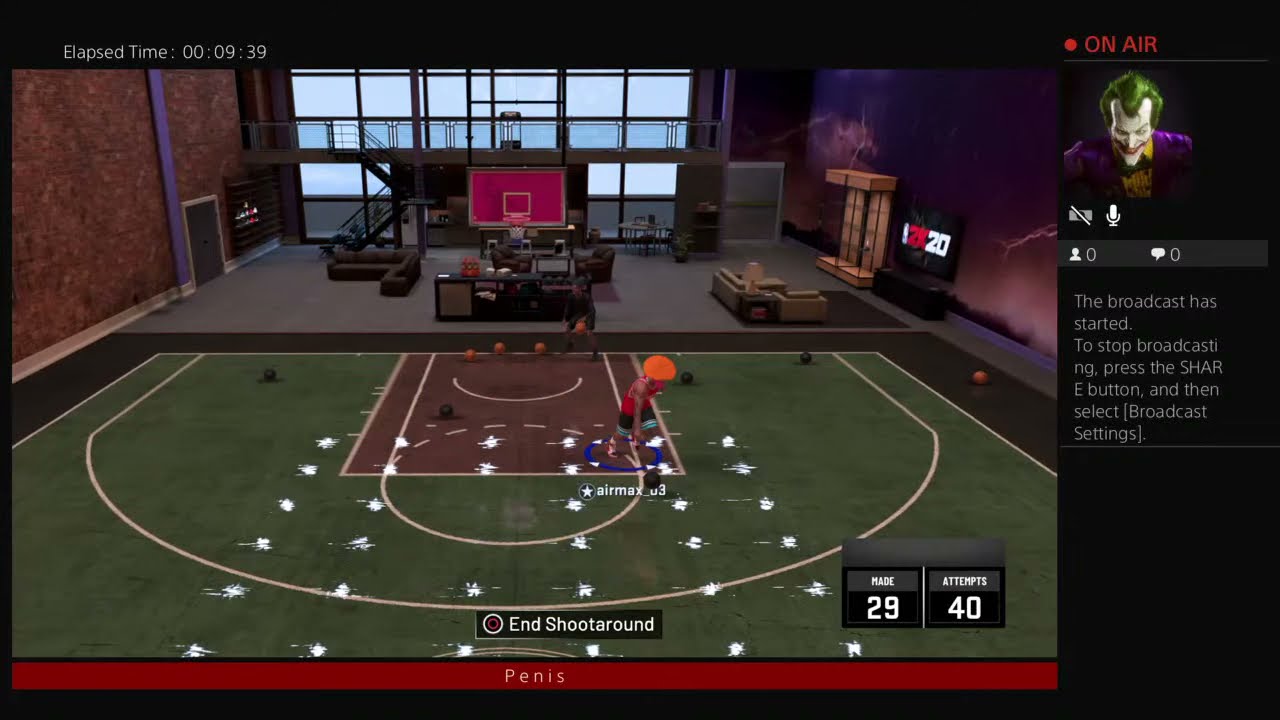This detailed screenshot captures the live-streamed gameplay of a basketball video game on a PlayStation console. The horizontal rectangular image primarily showcases a half basketball court on the right side, which is detailed with a circle, foul shot line, three-point line, and dark red foul areas. The red basket is prominently featured, and behind it is a peculiar lounge setting with industrial-style furniture and a large window, contrasting sharply with the sports environment.

The court itself is a mix of dark green and purple hues adorned with numerous white dots. In the center, a player, identified by their orange hat, red top, black, and green Air Max U3 shorts, is engaged in the game. The scoreboard displays made 29 versus attempts 40, while the bottom left corner bears the red banner notoriously labeled with "penis" in white text.

An overlay on the gameplay, marked by a black border on the top and right sides, provides streaming details. The upper edge shows an elapsed time of 9 minutes and 39 seconds. On the right, a red "on air" indicator is accompanied by the player's avatar, a Joker image from Batman, signifying zero spectators and zero comments. The bottom of the overlay instructs users on how to stop the broadcast via the share button, adding another layer to the streaming interface. The overall scene gives a surreal mix of casual gaming, a semi-professional sports setting, and home comfort, meticulously blending the virtual and real worlds.